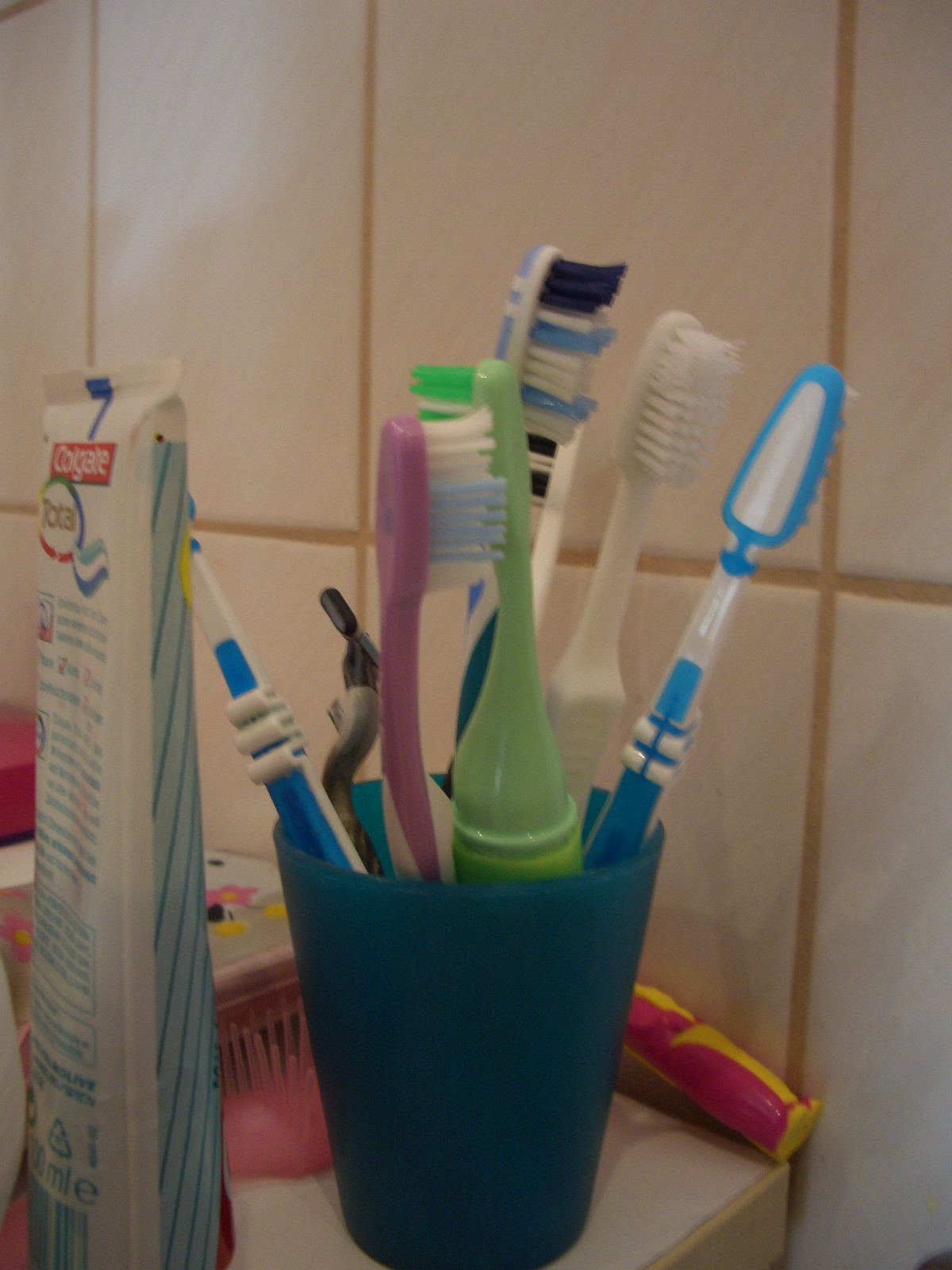In a close-up photograph taken in a bathroom against a backdrop of white grid tiles, a bright blue cup brimming with an array of colorful toothbrushes commands attention. This makeshift toothbrush holder contains six toothbrushes in various hues: a blue and white toothbrush, a lavender one, a chubby light green one, an all-white one, and another blue and white toothbrush laying on its side. Nestled nearby on the counter, a red and yellow child's toothbrush lies outside the cup. Beside the cup stands a tube of Colgate Total toothpaste, its trademark red-and-white design turned towards the camera. Additional bathroom items, like a small child's comb or brush, and hints of pink details, appear in the background, adding a lived-in and family-friendly feel to the scene, while the white tiles and beige grout create a clean, minimalist backdrop.